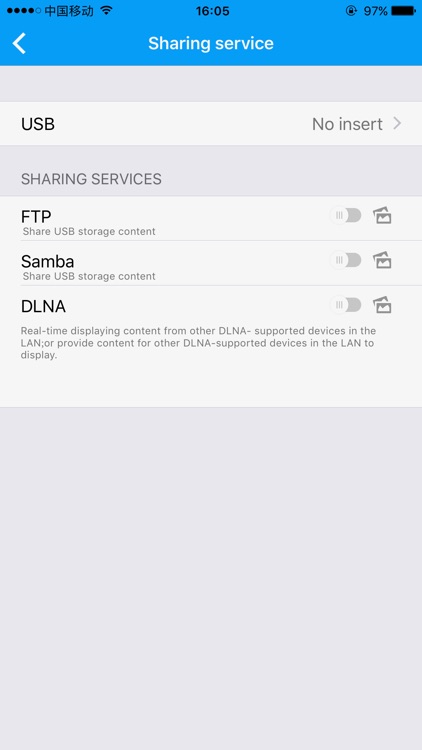Descriptive Caption:

"This is a detailed screenshot of a phone's interface captured at 16:05, displaying a comprehensive view of its file-sharing services. The top bar is a distinctive blue, housing a 'back' button overlaid with white text and iconography. It shows strong signal strength with four bars and full Wi-Fi connectivity. The phone's battery is notably charged at a healthy 97%. Below the 'Sharing Services' heading, written in Mandarin Chinese, various options are shown:

1. **USB** - Currently, no device is inserted.
2. **File Transfer Protocol (FTP)** - Option to share USB storage content is turned off.
3. **Samba** - Also set to off for sharing USB storage content.
4. **DLNA** - Details the ability to display real-time content to other DLNA-supported devices in the local area network (LAN) and vice versa.

The visual structure is complemented by a grey-silver area beneath these options, presenting an orderly and organized design. While the user conveys they were distracted by fireworks and a dog's bark, the screenshot effectively captures the core functionalities available in the 'Sharing Services' menu."